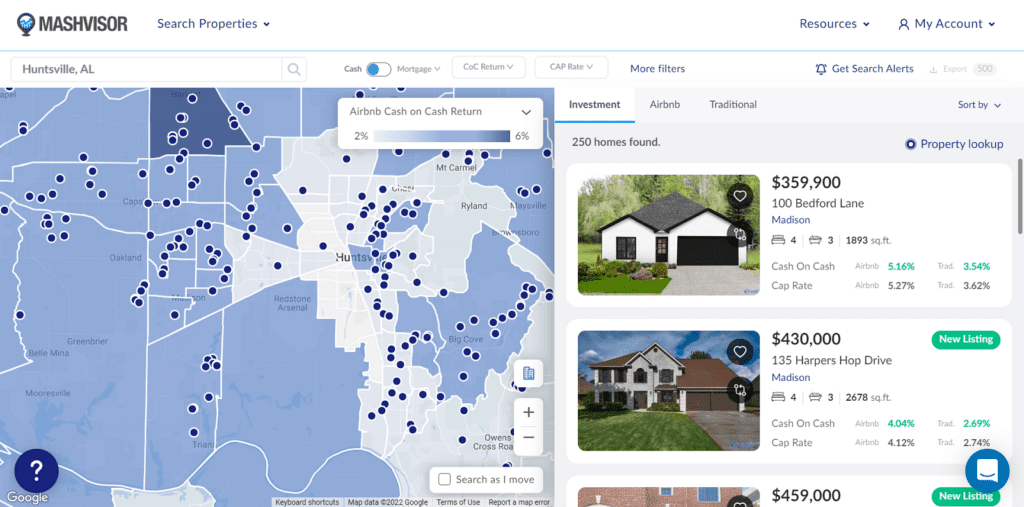The image is a detailed screenshot of a community-based real estate website. The top left corner features the website's logo, "MassVisor," in a dark black font, adjacent to a gray text reading "Search Properties." On the upper right side of the screen, navigation links for 'Resources' and 'My Account' are visible.

Centrally, a map with various shades of blue showcases locations related to "Airbnb cash on cash return" values, with numerous small blue dots scattered across it, indicating different properties. Two notable darker blue areas are noticeable to the left of the center on the map. At the bottom of the map, a small blue circle with a white question mark inside it serves as a help or information icon.

To the right of the map, the text "250 homes found" highlights the number of properties listed. Below this, there are thumbnail images and brief details of several properties: the first is a generic stock photo of a white house priced at $359,900, the second is a real photo of a two-story house priced at $430,000, and the third, which lacks clear details, is priced at $459,000. Additionally, on the far right bottom side of the screen, there is another blue circle containing a whitish-colored box, possibly indicating additional options or settings.